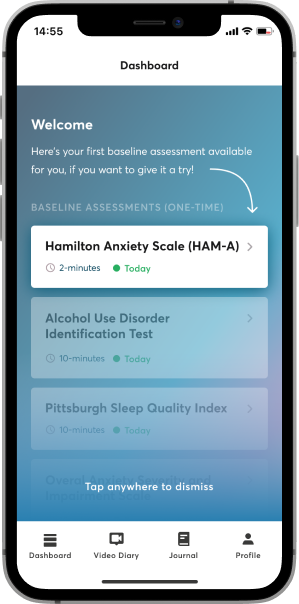A screenshot of a mobile wellbeing application is displayed on a phone, indicating the time as 14:55 (2:55 PM). The interface appears to be a dashboard, with the word “Dashboard” prominently shown in the center, accompanied by a greeting “Welcome.” The user is presented with their first baseline assessment for completion, outlined with the text: "Here is your first baseline assessment available for you. If you want to give it a try, baseline assessments one time."

The assessments listed include:

1. Hamilton Anxiety Scale (H-A-M-8) – taking approximately 2 minutes.
2. Alcohol Use Disorder Identification Test – estimated at 10 minutes.
3. Pittsburgh Sleep Quality Index – also about 10 minutes.

These options are emphasized in green for the current day's tasks. The design features a white, blue, and green color scheme, enhancing readability and user engagement.

Navigation options at the bottom of the screen are named: Dashboard, Video, Diary, Journal, and Profile, suggesting comprehensive tools for personal wellbeing tracking and management.